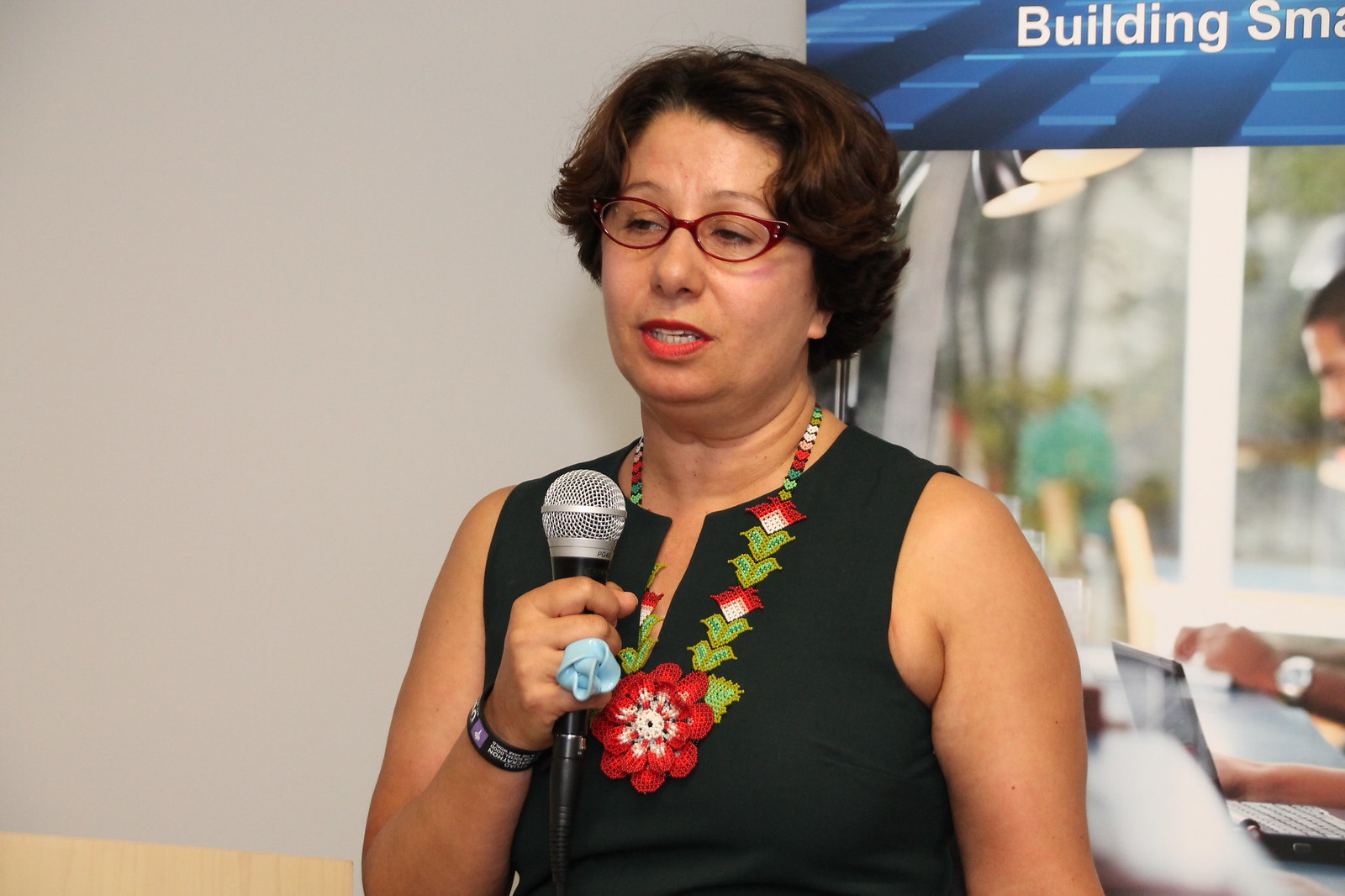In this full-color indoor seminar photograph, a middle-aged woman is seen standing and speaking into a silver microphone. She has short dark hair and is wearing distinctive red-rimmed glasses. Her outfit includes a blue top adorned with a colorful flower necklace, and she also wears a unique flower-shaped ring on her right ring finger. Positioned under a blue sign with white text that partially reads "Building Smart," the woman is engaged in delivering a speech. Behind her, there are lamps illuminating attendees working on computers, one of whom is visible in the background. The setting suggests a professional environment, possibly during a Q&A session, with a window faintly discernible along with the focused gentleman typing on his computer.